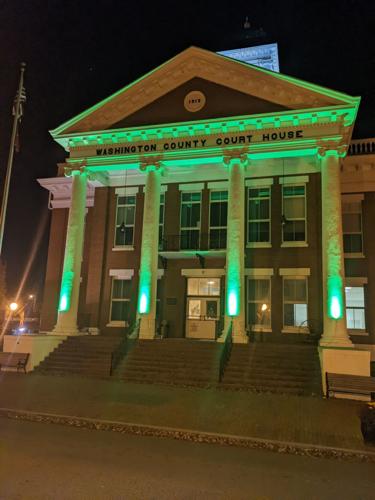The image captures a low-resolution, night-time photograph of the Washington County Courthouse, likely located in a smaller town. The courthouse features a prominent triangular frieze at its top, with "Washington County Courthouse" inscribed in black lettering. Four brightly lit ionic pillars, illuminated in a vivid lime green possibly for a Halloween theme, dominate its facade. The front-facing section also includes large, utilitarian windows suggestive of architecture from the 1920s to 1940s. The scene is further characterized by rusty brown steps leading up to the courthouse, and an American flag on a flagpole situated to the left. The courthouse’s tower is subtly accented with a bright blue light, contrasting with the intense green below. The photograph was taken in total darkness, with the courthouse appearing largely closed and unoccupied for the night.